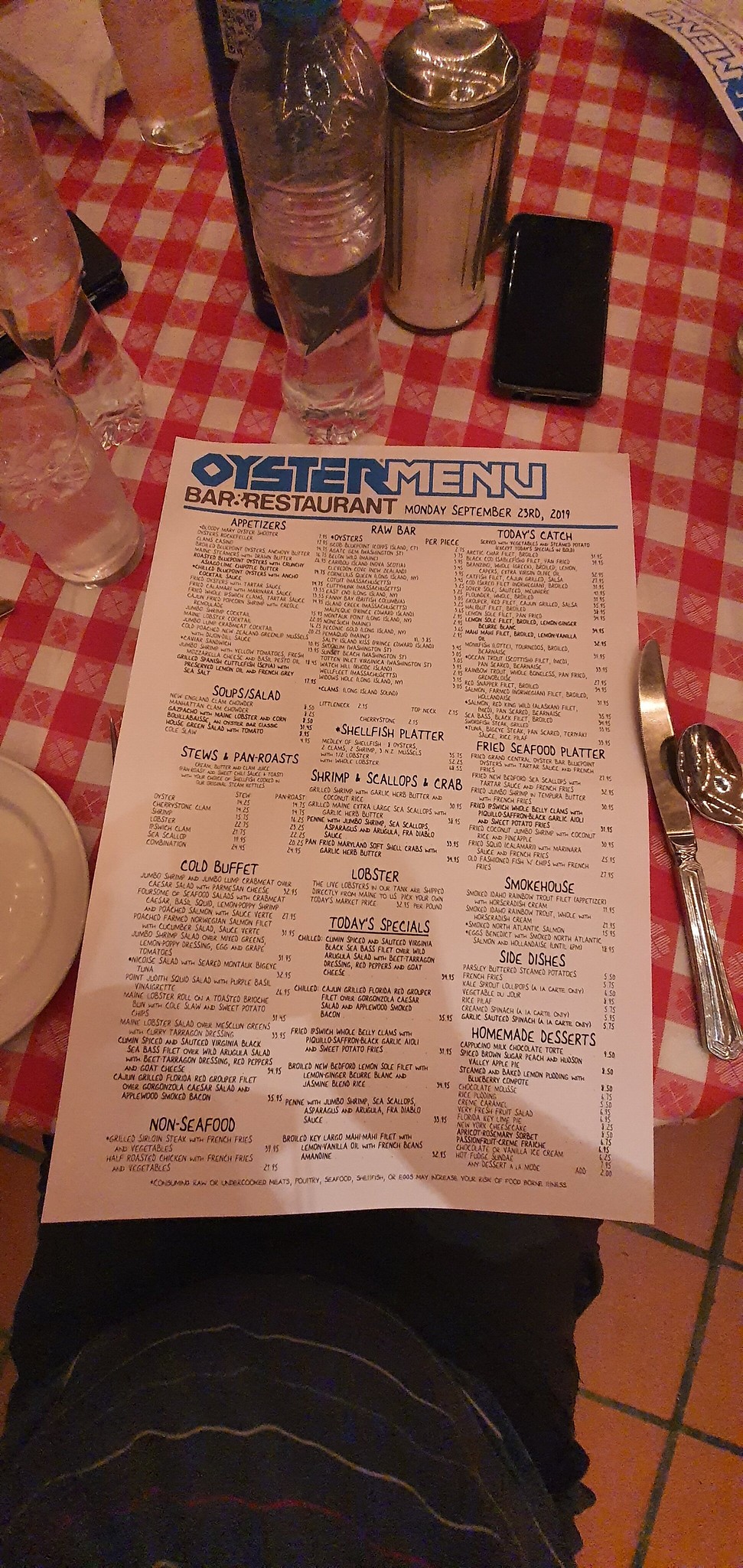This image captures an overhead view of a restaurant setting, centered around a single sheet of paper that serves as a menu. The top of the menu features the heading "Oyster Menu, Bar, Restaurant" with the word "oyster" prominently displayed in blue text. Although the page is filled with detailed information, the small font size renders it unreadable from this vantage point. 

Above the menu, three water bottles are visible—two positioned on the left and one situated directly above the menu. Adjacent to these is a sugar shaker and, to the right, the black phone of the person taking the photo, encased in a black cover. 

To the left of the menu, there is a portion of a small white plate, partially cropped out of the frame. On the right side, a butter knife and a spoon are laid out. The entire arrangement rests on a red-and-white checkered tablecloth, adding a rustic charm to the scene.

In the bottom right corner of the image, the floor is visible, characterized by white tiles with dark-colored grout. The lower part of the photo appears to show a person's body, though it's somewhat indistinct due to the dark clothing—likely black pants and a striped shirt.